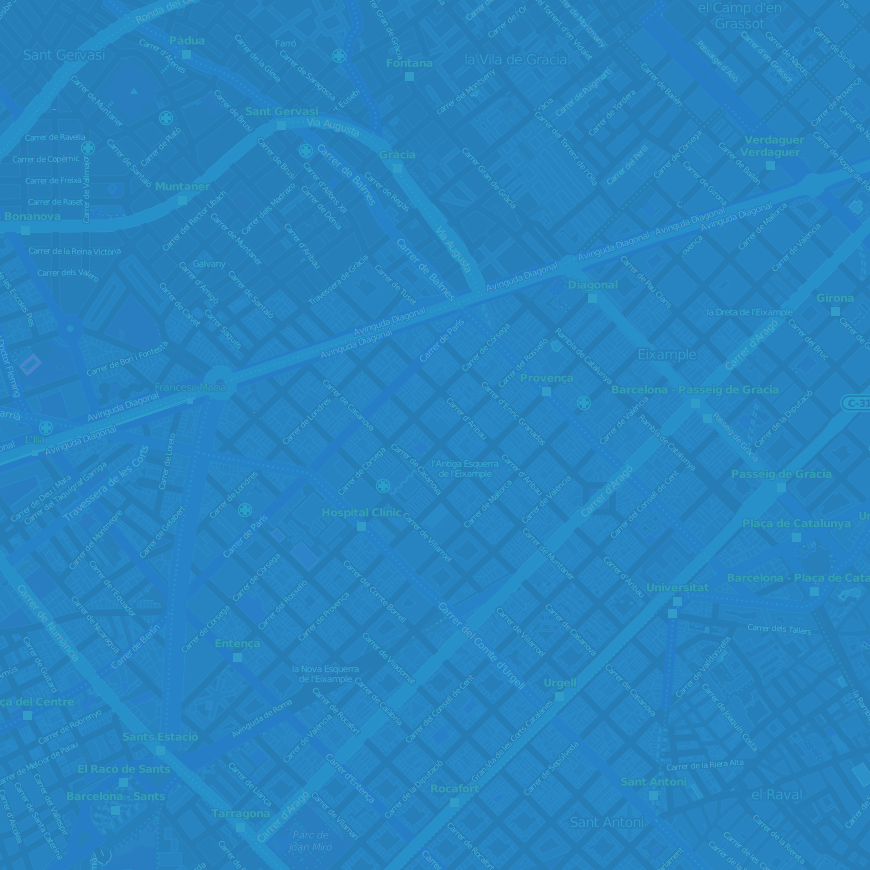This intricate map, rendered predominantly in shades of blue, provides a detailed aerial view of a city. Highlighted with labels in light white and green, the map demarcates various neighborhoods and key locations within the urban landscape. Notable landmarks include El Campton Resort and Hospital Clinic, though the lettering is quite small and challenging to read. 

The map features major roadways and a variety of buildings, meticulously outlined to offer a comprehensive guide to city navigation. Among the legible areas are Barcelona Place de Port Passa da Graça, St. Giovard, Fontana, La Villa de Graci, and St. Etombe, indicating distinct sections and neighborhoods within the city. The map appears to be in a non-English language, adding a layer of local authenticity to the depiction. Overall, this detailed city map serves as a visual tool for understanding the layout and divisions of this expansive urban area.